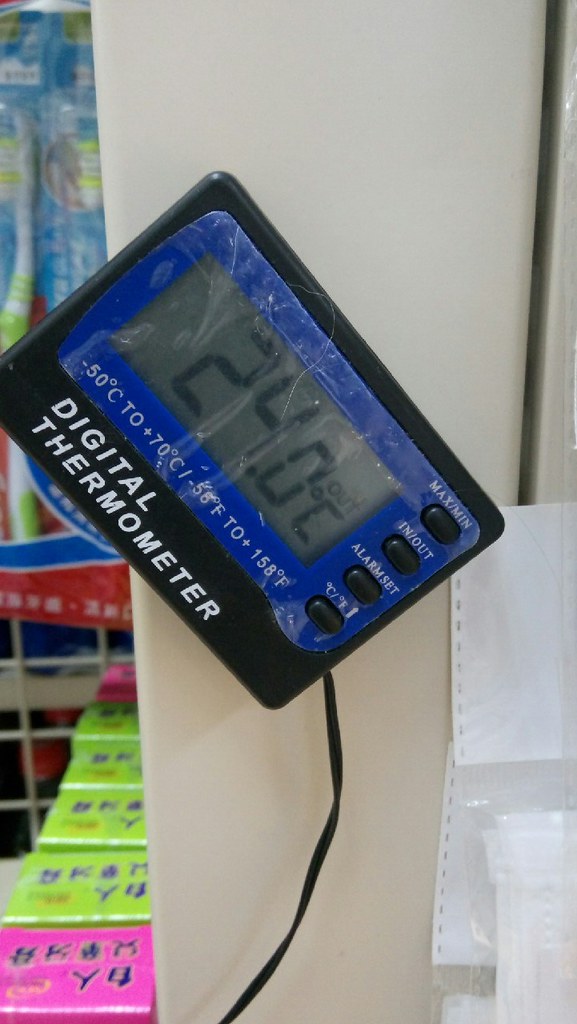This tall, narrow image prominently features a digital thermometer positioned centrally and facing upward. The thermometer's black background prominently displays "Digital Thermometer" in white lettering. A digital readout shows "24.0°C" beside the label "OUT", encased within a blue border that is outlined by a black frame. Below the displayed temperature, the measurement range "-50°C to +70°C / -58°F to +158°F" is indicated in white letters on a blue background.

To the right of the display, four black buttons with small white labels can be seen: "MAX/MIN" at the top, followed by "IN/OUT", "ALARM SET", and a fourth button with illegible text due to smudging. The thermometer appears to be affixed to a white wall, with a black wire extending from its bottom. Pieces of paper, possibly ripped from a spiral notebook, are taped next to the device on the wall.

In the distant left background of the image, there are glimpses of a store interior that includes shelves with a variety of products. Among these are boxes featuring Japanese script, including four yellow boxes and one pink box, suggesting the setting may be a retail store in Japan. The use of Celsius on the thermometer supports this inference, as the metric system is commonly used in Japan.